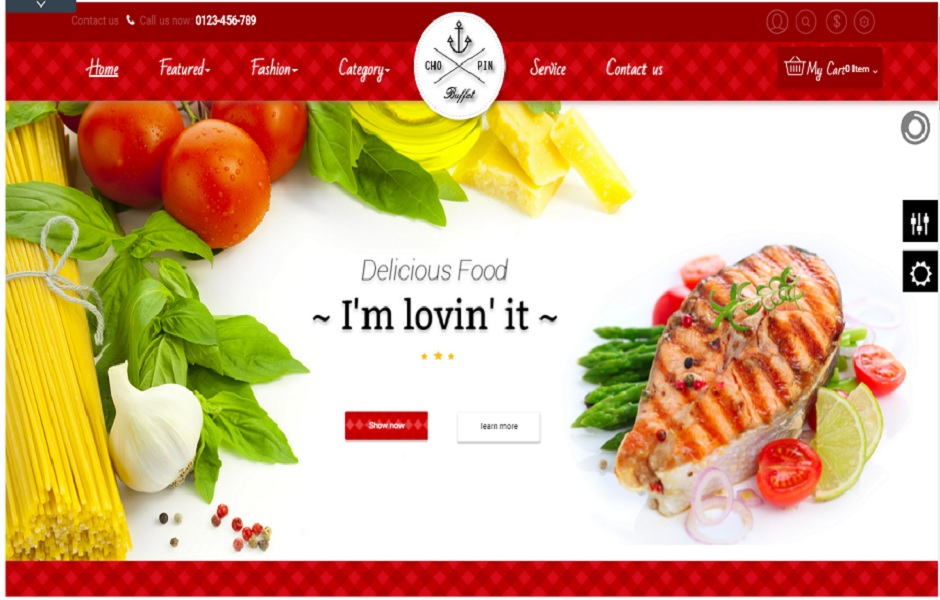The webpage features a predominantly red and white background. At the top, there's a red banner with "Contact Us: Call Us Now at 0123456789" in white text on the left side. Directly below this, navigation links labeled "Home," "Featured," "Fashion," and "Category" are displayed. 

Centered in the header, a white logo with black accents depicts a unique symbol: a black "X" with an anchor at the top, a chow at the left, a pin at the right, and a buffet at the bottom. On the right side of the banner, white text reads "Service," "Contact Us," with a drop-down button labeled "My Cart (0 items)" in white.

The main section of the webpage has a white background showcasing various food items. To the left, a bundle of uncooked spaghetti is neatly tied with white thread, accompanied by a large, whole garlic clove beneath it, surrounded by several basil leaves and three tomatoes. Scattered around are greens and what appears to be yellow fruits. 

At the bottom left, there’s a grilled filet of fish artfully presented with lime wedges, tomatoes, and asparagus. Centrally positioned black text announces "Delicious Food—I'm Loving It" with two buttons below: a red "Shop Now" button and a white "Learn More" button with black text. The bottom of the page is capped with a thin red strip, completing the design.